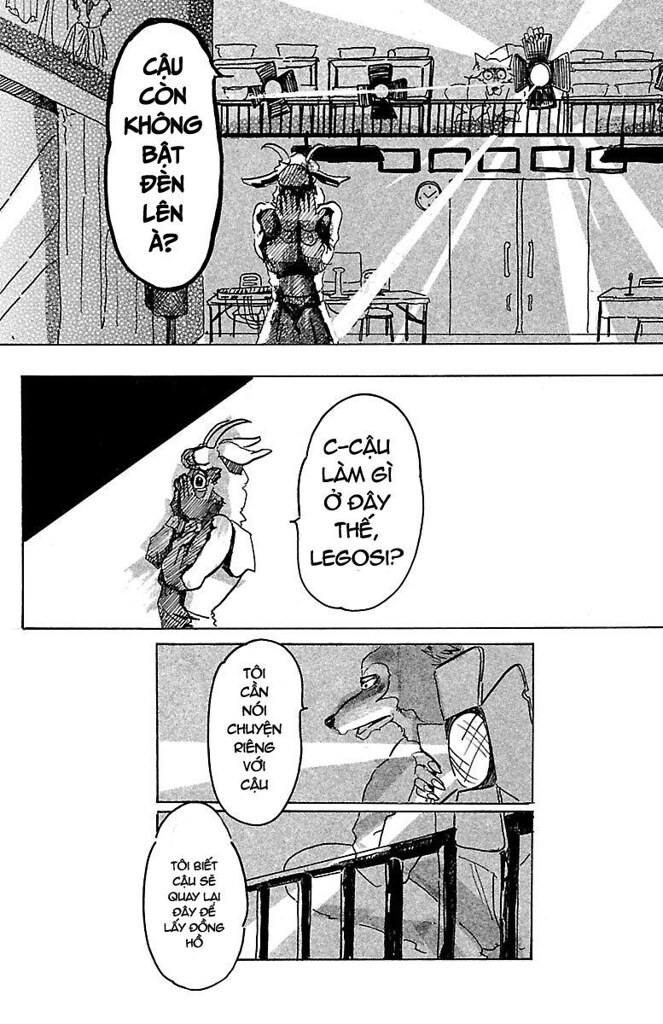This detailed comic strip comprises three hand-drawn, black-and-white panels, each meticulously illustrating a scene that merges surreal characters with a touch of theatrical drama. The top panel presents a distraught minotaur-like creature, sitting with its hands covering its face, as if crying, situated in a setting that resembles a movie theater or a stage with doors behind it. Above this sombre figure, on a higher level, a fox-like or raccoon-like animal operates what seems to be a spotlight, casting a beam onto the scene below.

The central and lower panels reveal more about these two characters and their peculiar interactions. The central panel provides a side view of the minotaur or goat-like creature, still in a tearful pose, with foreign text in a speech bubble emanating from it, suggesting a dialogue or inner monologue that is integral to understanding the scene but remains cryptic due to its unfamiliar language, possibly Filipino.

In the final panel, the spotlight operator is given more focus, showing the creature squatting while manoeuvring the light source, with additional foreign text ciphered within speech bubbles, adding to the intrigue. Despite repeated attempts to decipher the characters, the exact nature of the dialogue remains elusive, further mystifying this enthralling comic strip. The detailed artistry of the animals and the thoughtful layout highlight the melancholic yet captivating storyline that transcends the language barrier.